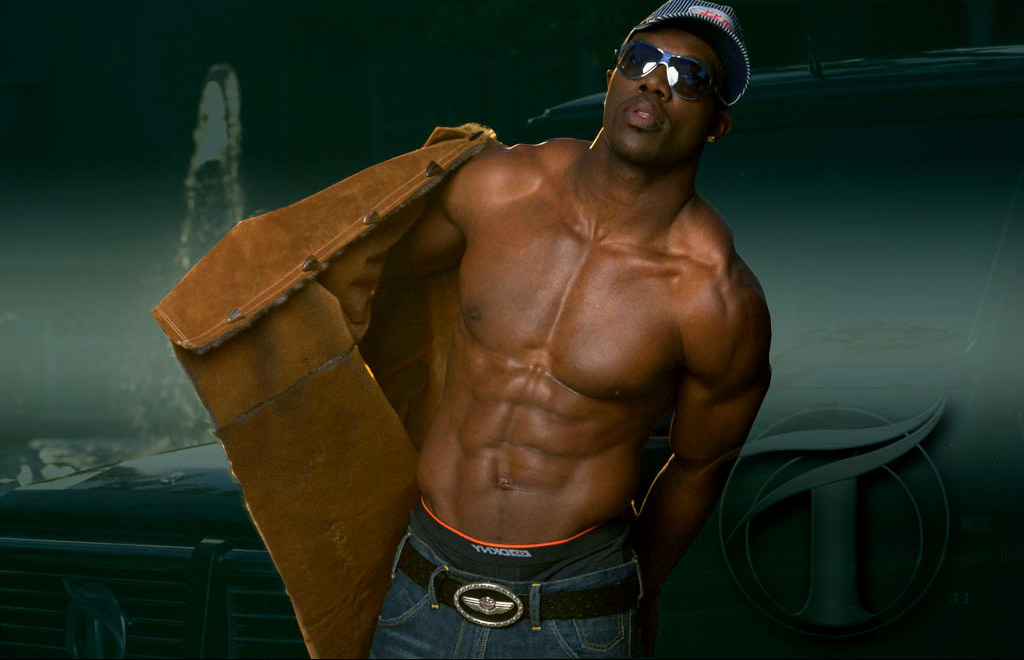In this image, a shirtless man with dark skin is captured in a staged scene suggestive of an artistic photoshoot or video recording session. He's dressed in blue jeans secured by a black belt with a silver buckle, and part of his underwear is visible above the jeans' waistband. He complements his look with dark sunglasses and a blue striped baseball cap, and appears to be either wearing or carrying a brown jacket slung over his shoulder. The man also seems to be wearing earrings. The backdrop of the image is predominantly gray, and a car is faintly visible behind him. The bottom right corner features a distinctive logo resembling a tilted, leafy cross 'T'. The overall palette of the photograph is muted, comprising primarily of browns, blacks, and dark blues, adding to the dramatic and stylized atmosphere of the scene.